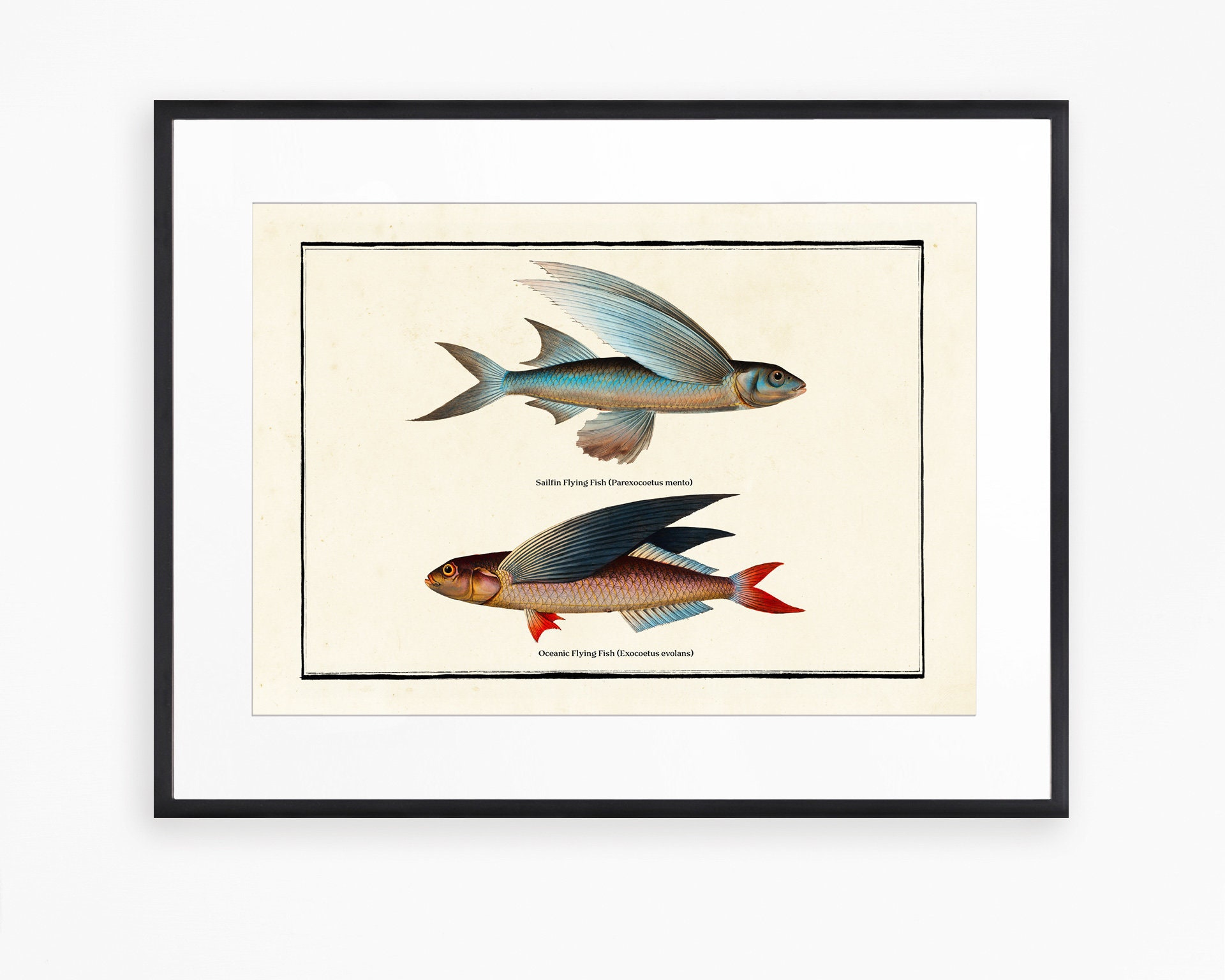The artwork is a framed painting of two intricately drawn flying fish displayed on a white wall. The painting is presented in a thin black frame complemented by a thick white mat, with the fish depicted on cream-colored, manila-like paper. A delicate black border encapsulates the fish, adding contrast to the soft background. 

The top fish, elegant and striking, is a turquoise with brown at the bottom, featuring elaborate turquoise fins and gills, resembling wings. Its side view shows a turquoise face with detailed eye depiction. The bottom fish, sturdier and bold, is a reddish-gold with blue accents, including large dark blue fins and wings. The scientific names of the fish are subtly inscribed beneath them, with the top fish titled as a "Silphian Flying Fish" and the bottom as the "Oceanic Flying Fish." This detailed composition combines fine art and scientific illustration, making it a captivating piece for any wall.